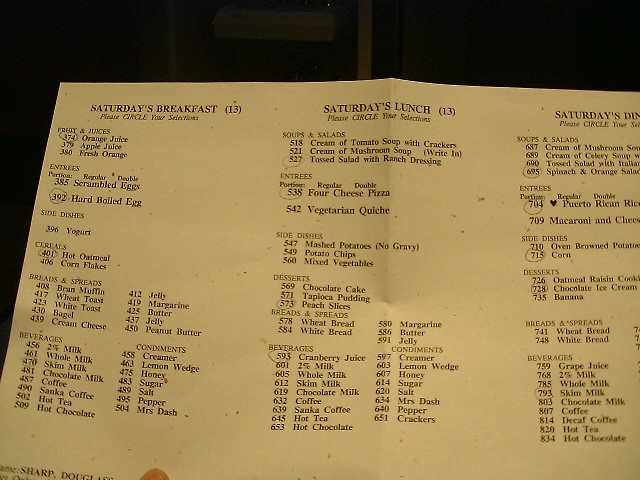The image features a menu set against a black or dark background, which may either be due to low lighting or the absence of any background elements. The document itself is a horizontal rectangle, and it appears to be a realistic photograph or possibly a scan. There is a hint of a finger visible at the bottom left, suggesting that someone is holding the menu.

The menu is printed on a white or slightly off-white page, with the text presented in black ink. The shading and lighting make the page appear a bit darker than it might actually be. The content is organized into three columns:

1. **Saturday's Breakfast** (left column) 
   - **Fruits and Juices**: 
     - 374 Orange Juice
     - 379 Apple Juice
     - 380 Fresh Orange
   - **Cereals**:
     - 401 Hot Oatmeal
     - 406 Corn Flakes

2. **Saturday's Lunch** (center column) 
   - **Entrees**:
     - 538 Four-Cheese Pizza
   - **Desserts**:
     - 569 Chocolate Cake

3. **Saturday's Dinner** (right column) - Partially cut-off 
   - **Breads and Spreads**:
     - 741 Wheat Bread
   - **Beverages**:
     - 759 Grape Juice

The menu items are listed with numbers ranging from 374 to 834, with the lowest number found at the top left and the highest at the bottom left. The detailed listing of food items includes a variety of breakfast options, lunch entrees, and dinner choices, providing a clear and structured overview of meal offerings for Saturday.